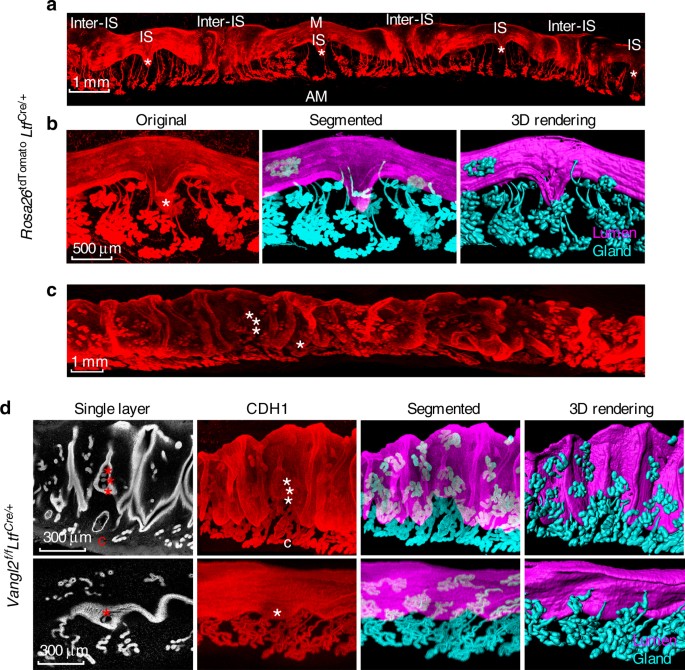This detailed color image predominantly features a scientific analysis of a biological specimen, likely highly magnified. The image is arranged in multiple rows and sections labeled A, B, C, and D, each depicting different stages of observation: original, segmented, and 3D rendering.

- **Row A** presents a single long red strip on a black background labeled as "original," "segmented," and "3D rendering." The red strip stretches from left to right, and beneath the top layer, there are vertical extensions resembling plant stems or branches, likely indicating some biological life-form.
  
- **Row B** drills down further, showing three images labeled "original," "segmented," and "3D rendering" of the same red object on a black background. The segmented view converts the red object into a purple top layer with blue-green extensions, almost like leaves on stems. This row includes a scale bar indicating 500 micrometers.

- **Row C** displays another red strip on a black background, segmented into detailed, high-magnification view labeled with one millimeter increments. This corresponds visually to what is observed in Row A.

- **Row D** consists of two sets of images on the left, labeled as 300 micrometers each. This section also follows the pattern of "original," "segmented," and "3D rendering." Here the object, CDH1, is shown in red on a black background, with the segmented and 3D rendering views emphasizing finer details of the subject.

Overall, the image uses bright colors to highlight the structures against a stark black background, aiding in identifying specific biological features, such as possibly a type of gland or cellular structure, with detailed legends and scales to illustrate the magnification levels.